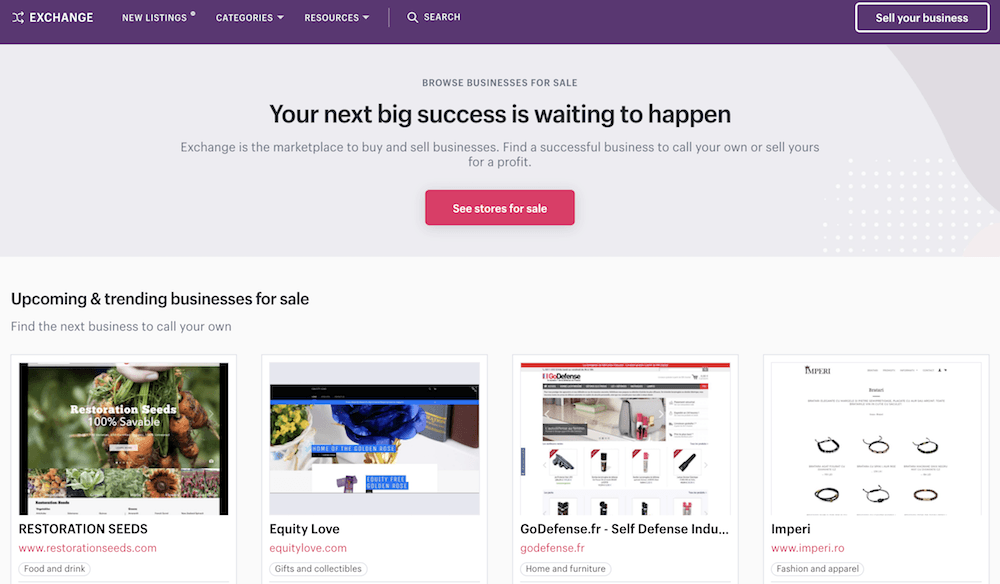### Screenshot Description of Online Business Marketplace Interface

**Top Navigation Bar**:
- **Exchange**: Located at the top left-hand corner, featuring two crossing arrows icon.
- **New Listings**: Positioned next to "Exchange".
- **Categories**: Includes a drop-down arrow, denoted by a dot separator.
- **Resources**: Features a drop-down arrow, followed by a vertical line.
- **Search Bar**: Accompanied by a magnifying glass icon.
- **Sell Your Business**: A white-bordered box on the far right of the navigation, all elements are displayed in purple.

**Main Header**:
- Background color: Gray.
- Header Text: 
  - **Primary Text**: “Browse Businesses for Sale”
  - **Secondary Text**: "Your Next Big Success is Waiting to Happen" in large black font.
  - **Description**: "Exchange is the Marketplace to Buy and Sell Businesses. Find a successful business to call your own or sell yours for a profit," in gray font.

**Highlighted Section**:
- **Prominent Feature**:
  - Red box labelled “C-Stores for Sale”.
  - Accompanied by white dots on the right and a dark gray wave-patterned triangle.

**Upcoming and Trending Businesses**:
- Displays in a lighter gray background with the title "Upcoming and Trending Businesses for Sale. Find the next business to call your own."

**Business Listings**:
1. **Restoration Seeds**:
   - Image: Large picture of carrots and carrot leaves, smaller images include a sunflower, two leaves, another bunch of carrots, and flowers.
   - Text: "Restoration Seeds"
   - URL: In red, "www.restorationseeds.com"
   - Category: White oval with "Food and Drink".

2. **Equity Love**:
   - Image: Blue flower with gold stems next to yellow potted flowers.
   - Text: "Equity Love"
   - URL: In red, "www.equitylove.com"
   - Category: White oval with "Gifts and Collectibles".

3. **GoDefense**:
   - Image: Showcasing a gun, flashlight, mace, and a gray bag with cans of mace in front.
   - Text: "GoDefense"
   - URL: In red, "www.godefense.fr"
   - Category: White oval with "Home and Furniture".

4. **Empiri**:
   - Image: Indistinct items resembling necklaces or stethoscopes.
   - Text: "Empiri"
   - URL: In red, "www.empiri.ro"
   - Category: White oval with "Fashion and Apparel".

This cleaned-up and detailed description paints a clear picture of the visual and textual elements in the screenshot, making the structure and content of the marketplace interface easy to understand.